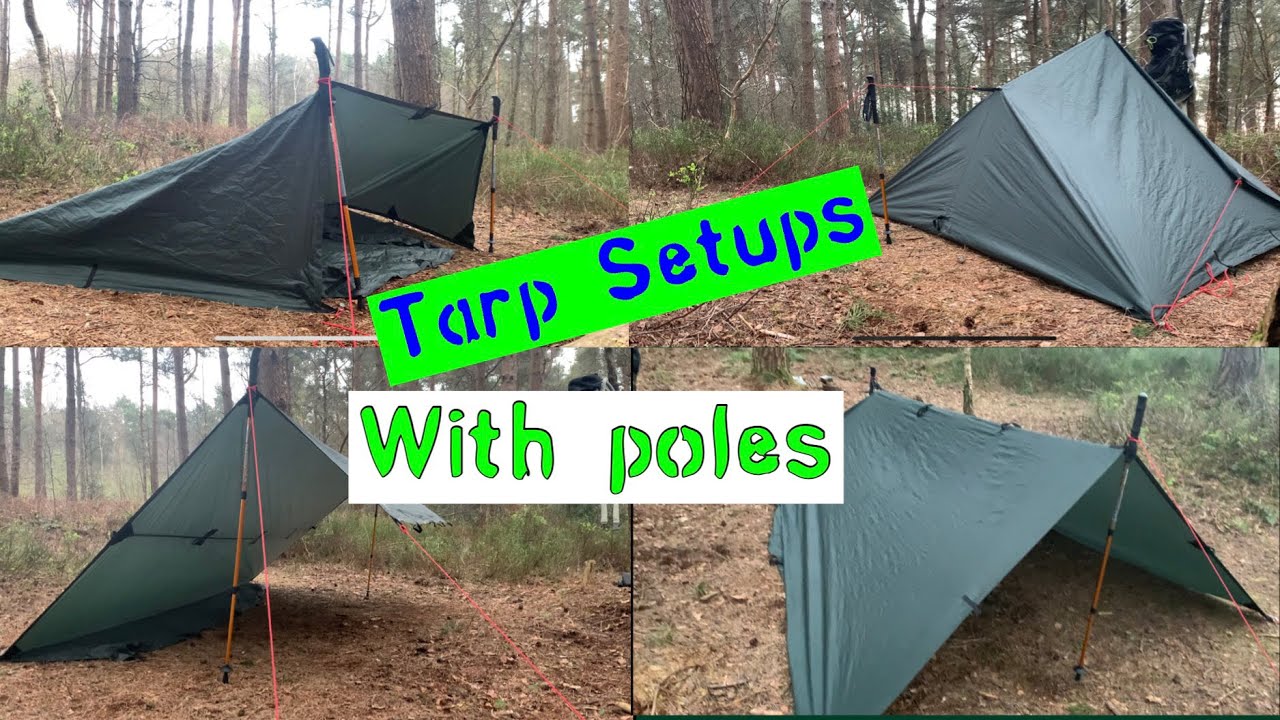The image is a composite of four sequential color photographs, arranged in a 2x2 layout against a forested backdrop. Each photograph depicts various configurations of a dark green tarp used to set up tents. The top left photograph shows a tarp with a square opening facing right, suggesting an entrance. The top right photograph features a triangular tent formed by folding the tarp on three sides. The bottom left image displays a lean-to setup, creating a shed-like structure, while the bottom right shows an open-front tent held up by a hiking stick in the center. The ground is a mix of brown mulch, dirt with green grass, and shrubs, surrounded by trees with brown bark, indicating a woodland environment. Overlaid on the center of the image are two horizontal rectangles with text. The top rectangle is tilted, lime green in color, with the blue stenciled text "tarp setups." Below it, a white rectangle holds the lime green text "with poles." The sky in the background is dull and hazy, adding to the dense forest atmosphere. The tents, anchored by metal poles—orange and pink—and pink string tied to ground stakes, illustrate different ways to configure tarp setups in the outdoors.